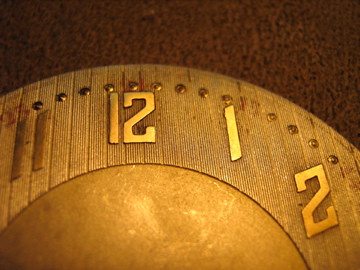This color photograph captures the top right section of a handcrafted wall clock, framed against a speckled brown and dark-patterned background, possibly a rug or wallpaper. The clock itself appears to be made of richly textured wood with a smooth, gold-toned plate at its center. The visible portion includes golden, analog numbers 11, 12, 1, and 2, each accompanied by small golden studs spaced closely above them. The light is focused on the clock, emphasizing the golden shine of the numbers and the detailed wood design, while the hands of the clock are not visible. Only about one-third of the clock is shown in this horizontally oriented, rectangular image.